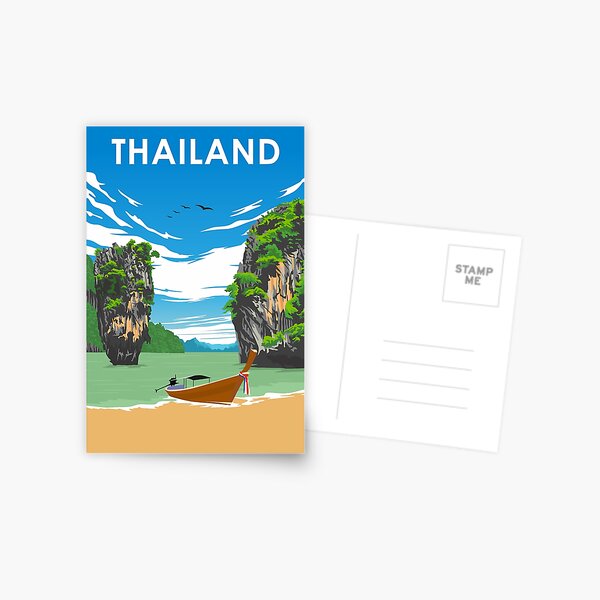The postcard from Thailand features a vibrant scene with "Thailand" prominently displayed in thin, white capital letters at the top against a clear blue sky adorned with wispy clouds and four birds. In the foreground, a brown canoe with a red, white, and blue ribbon is positioned at the edge of a sandy beach, near greenish waters. Tall, narrow rock formations with lush trees rise from the water, resembling mini plateaus. In the background, a majestic mountain range and additional tree-covered areas complete the picturesque vista. The postcard's reverse side is blank, with designated spaces for a stamp and four lines for writing. This visually stunning postcard impeccably captures the essence of a serene Thai vacation getaway.